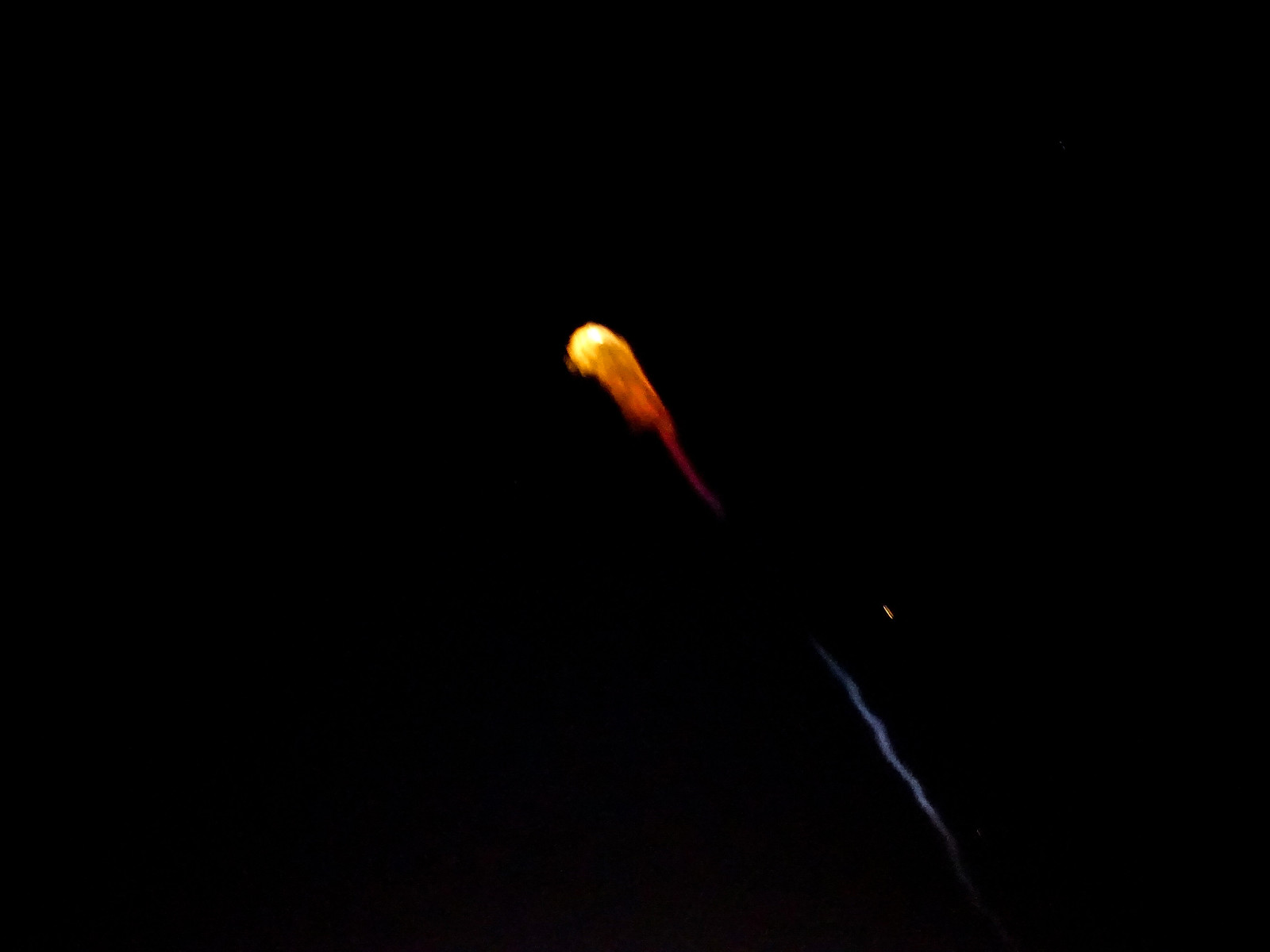The image captures a striking moment of a shooting star streaking across a slightly darkened sky, perfectly timed by the photographer. The sky serves as a nearly black background, which heightens the dramatic effect of the celestial event. The center of the photo features a brilliant yellow and orange fireball moving upward and to the left, with a rounded head that flares out in waves of vibrant, fiery colors. A trail follows this fireball down and to the right, transforming from orange to a dark blue or bluish-gray hue that extends almost to the bottom of the image. Within this smoky, trailing tail, a small speck of yellow can be seen, possibly indicating a fragment breaking off from the main meteor. The interplay of colors—yellow, orange, and blue—against the dark backdrop creates a visually stunning and dynamic display of a meteor in motion.